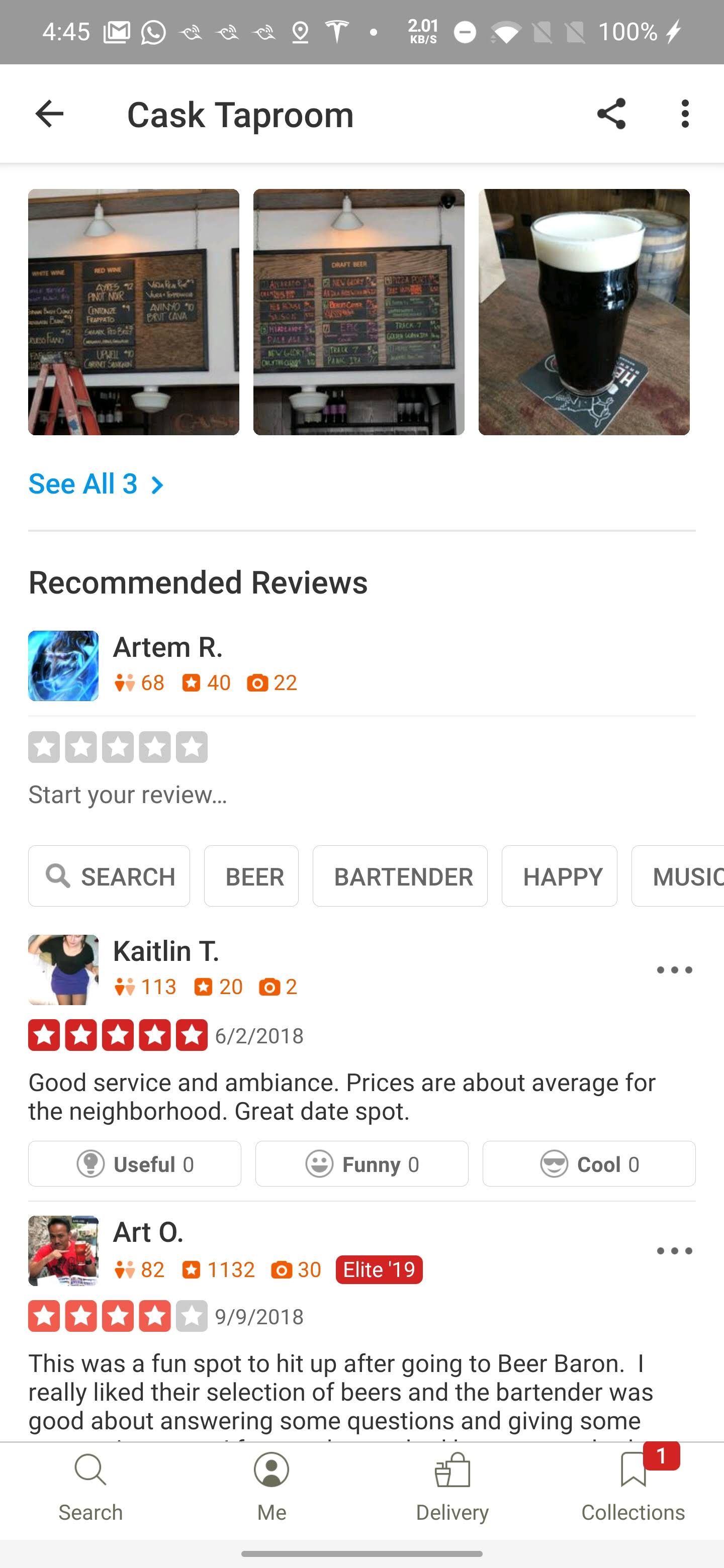This image is a smartphone screenshot taken at 4:45 PM, with the battery fully charged at 100%, and a strong signal indicated. The interface is displayed against a white background and features the text "CASKAPROM" with an arrow pointing to the left. On the right side, three vertical dots are visible, likely representing a menu or additional options. 

Centering on the screen are images showcasing various beers and food items, illustrating a strong focus on the beer selection. 

Just below the images, the text "Recommended Reviews" appears, followed by the prompt "Start your review."

The first review is by Caitlyn, who rated the place five stars, mentioning, "Good service and ambience. Prices are above average for the neighborhood, but it's a great date spot." Notably, her review has no votes for being useful, funny, or cool.

The second review is by Art O, who awarded four stars. His review states, "This was a fun spot to hit up after going to Beer Baron. I really liked their selection of beers, and the bartender was good about answering some questions and giving some," but the review is cut off before it finishes.

At the bottom of the screen, navigation options include "Search," "Me," "Delivery," and "Collections," indicating different sections of the app or platform being used.